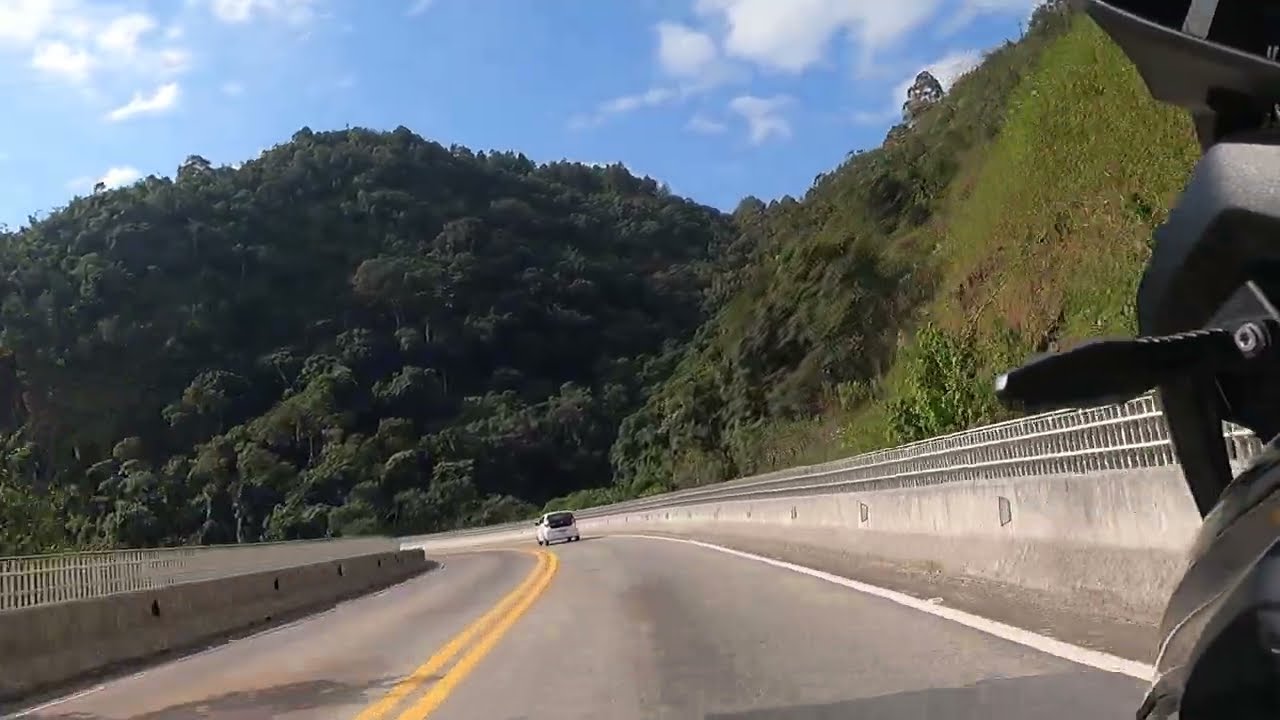The image captures a picturesque stretch of a two-lane highway bordered by gray concrete barriers on both sides. Dominating the center of the photograph is a long, winding road that leads to a distant white car, which is beginning to curve left. The point of view suggests the photograph was taken from a motorcycle, hinted at by the partial, black and gray silhouette of motorcycle components along the right edge of the frame. The road stretches straight ahead before disappearing into the lush, green hills that rise prominently in the background. These hills are teeming with dark green trees and bushes, with one large mound to the left and another overlapping it slightly to the right, extending out of the frame.

Above, the sky is a clear light blue, dotted with a few clusters of white clouds, primarily concentrated in the upper left and middle of the image. The sun, inferred from the light, appears to be shining from the left side, casting soft shadows. The overall composition blends the structured elements of the road with the natural beauty of the verdant hills and serene sky, creating a balanced and engaging scene.